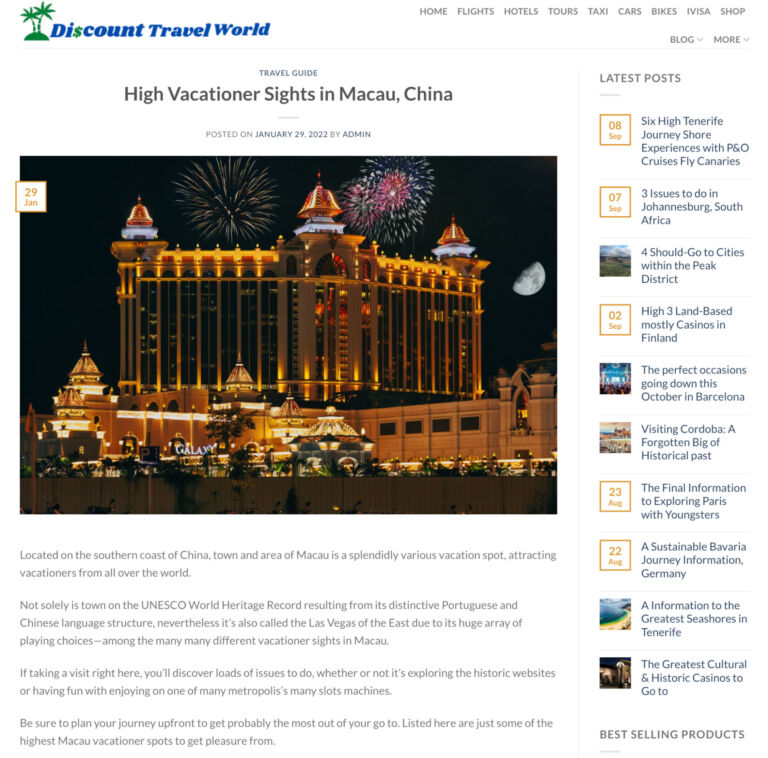This image captures a detailed view of a web page from Discount Travel World, a travel guide website. The headline of the page prominently reads "High Vacationer Sites in Macau, China," with the words "Travel Guide" in uppercase grey letters above it. The article was posted on January 29, 2022, by Admin.

The main visual element is a nighttime image of a grand palace illuminated with golden lights, accentuated by a stunning display of fireworks bursting in the sky above. The moon can be seen in the background, adding to the majestic atmosphere of the scene, which resembles an amusement park.

Below the image, the article begins with a description of Macau, highlighting its position on the southern coast of China and its recognition as a UNESCO World Heritage site due to its unique blend of Portuguese and Chinese architecture. The text aims to emphasize Macau’s appeal as a diverse vacation destination that attracts tourists from around the globe, although it contains some nonsensical language.

On the right-hand side of the web page, a sidebar lists the latest posts, featuring several other travel articles. At the top of the page, the navigation bar offers links to various sections of the site, including Home, Flights, Hotels, Tours, Taxi, Cars, Bikes, Visa, and Shop. This structured layout ensures easy access to a variety of travel services and information.